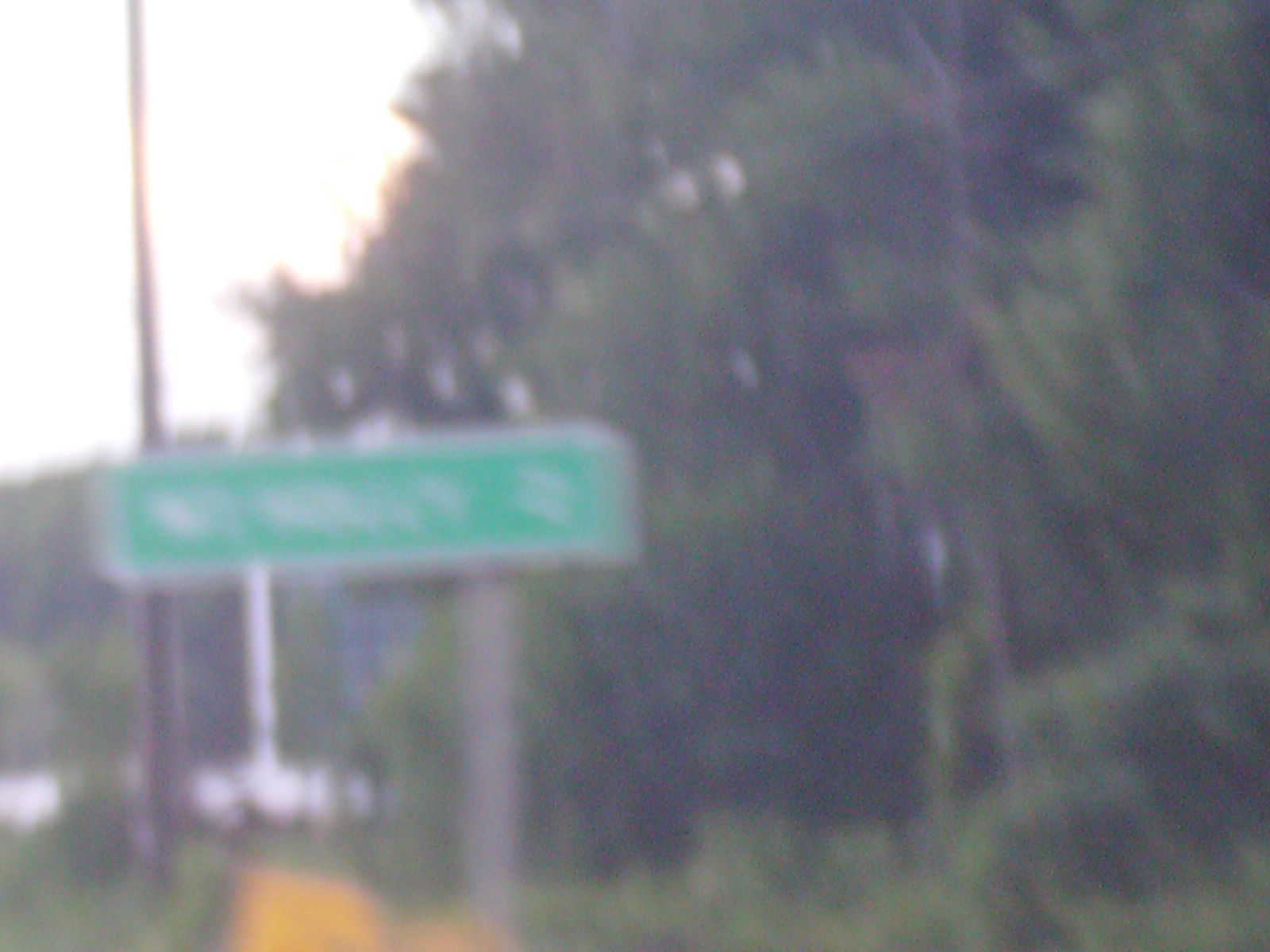The image exhibits a slightly blurry background with a prominent metal pole on the left side. The right side of the image is dominated by green leaves, presenting a lush, natural element. A green sign with some text is visible in the foreground, held up by another metal pole that is located towards the bottom left of the frame. The base of this pole appears to be yellow. The backdrop features a white area which might be part of the sky or another object. At the top left, the sky itself seems to be white, intersected by a wire that stretches across the frame. The overall composition contrasts industrial elements with natural foliage, creating a diverse and somewhat chaotic scene.